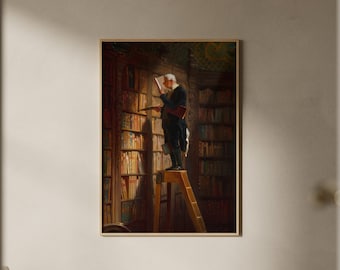The image depicts a painting hanging on a white wall. The painting captures a serene library scene, featuring an older man standing on top of a wooden stepladder. The library is filled with towering bookshelves, four of which are visible, each packed with numerous books across seven shelves. The man, illuminated by a sunbeam, appears to be deeply engrossed in reading a book he's selected. Dressed in an all-black suit with trousers, black shoes, and a white shirt, his gray hair and refined demeanor add to the scholarly atmosphere. The detailed brushwork and composition suggest it is likely an oil painting rather than a photograph.